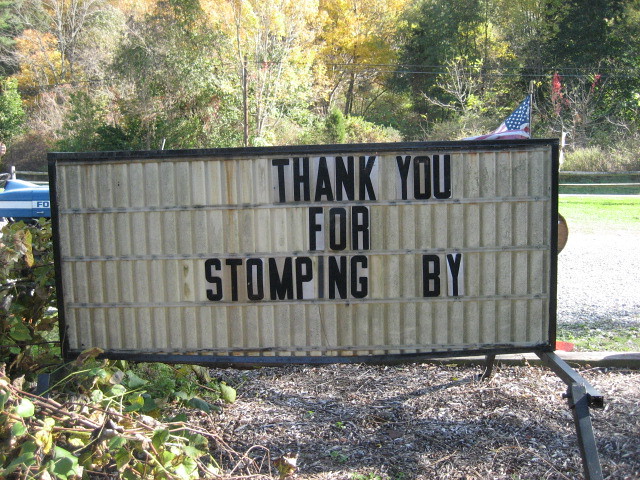In this color photograph taken in a natural outdoor setting, a prominent sign with a black metal frame and a tan or off-white background bears the message, "Thank you for stomping by" in black print. The sign is placed within a mulched landscape bed, surrounded by branches and green leaves, with additional brush and greenery visible on the left. An American flag mounted on a pole is situated behind the sign, partially visible against a backdrop of a stone path and a mix of trees displaying green, yellow, and occasional red leaves. In the distance, power lines can also be seen, adding to the scene's rustic ambiance. The composition suggests the sign might be part of a walking trail or park area, designed to bid farewell to visitors as they depart.